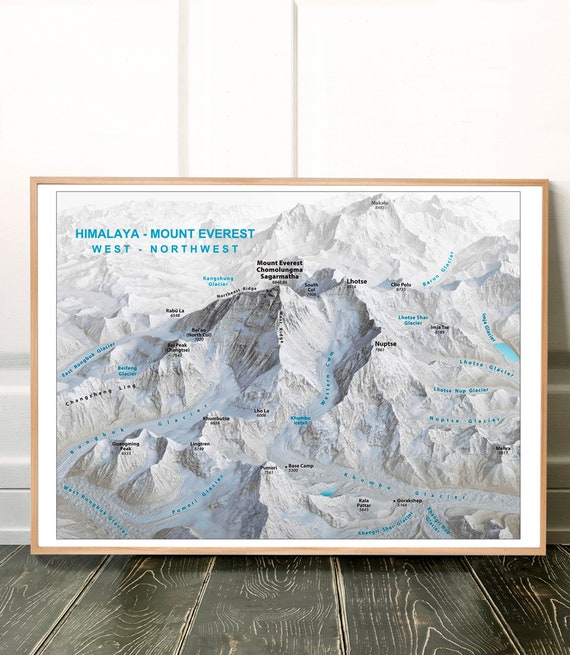The image depicts a detailed map of the Himalayas, prominently featuring Mount Everest. The map is framed by a light brown border and includes intricate trails and various peaks and valleys. The top-left corner of the map bears the blue text "Himalaya, Mount Everest" with "West, Northwest" written below it. The map, resting against a white-paneled wall, sits on a sleek, black-stained wooden floor accented with white crevices.